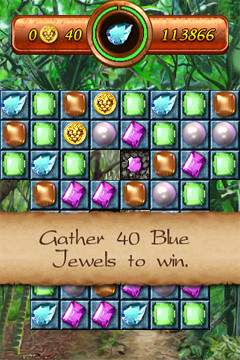The screenshot depicts an in-game interface with a top banner in a rustic red color displaying text in gold letters. At the top left, the banner reads "0," followed by a small circle, then "40," and on the right side, it displays "113866." In the center of the screen, there is a larger circle divided into a quadrant of rust color, chartreuse green, and black, with a diamond shape situated in the middle. The background features a lush green leafy motif.

At the bottom, a tan strip spans the lower third of the screen, containing an instruction: "Gather 40 blue jewels to win." The game grid, consisting of 8 columns across and 6 rows down, is filled with various-colored jewels, which include shades of blue, green, rust, gold, lilac, light lilac, and black.